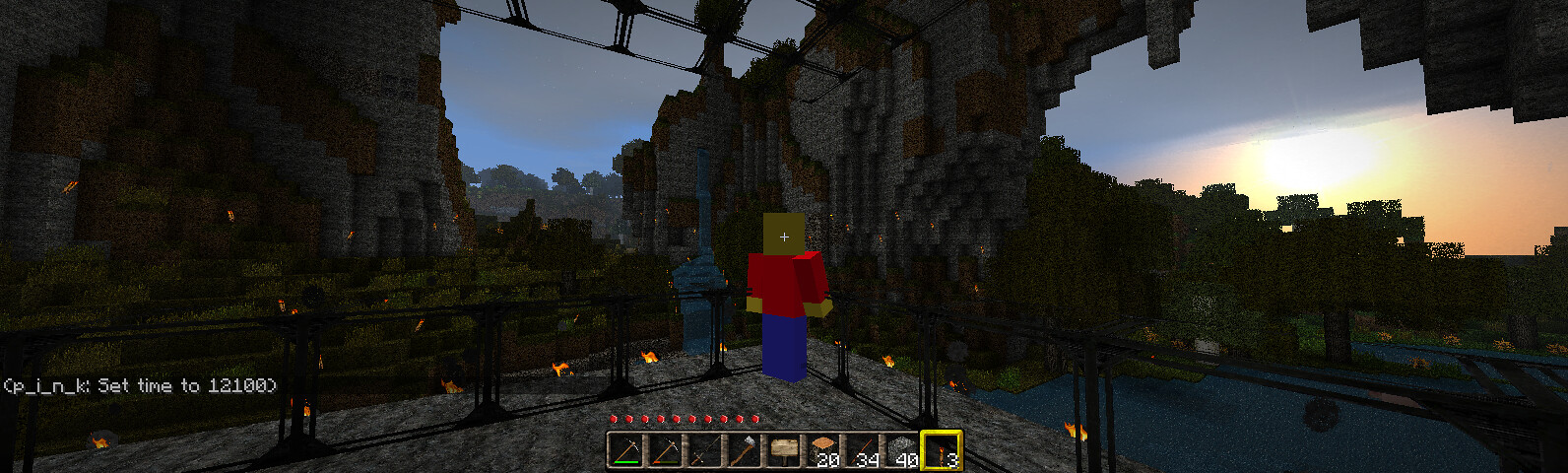This is a screenshot from the video game Minecraft, evident from the blocky, square terrain and features that are characteristic of the game. At the center of the image is the main character, customized with a skin different from the default Minecraft Steve, wearing a bright red long-sleeve shirt and blue pants. The character, with yellow hands and a brown, square-shaped head, resembles a Lego figure due to their boxy and rectangular appearance. The character is standing on a flat terrain, possibly on top of a constructed structure, encircled by lit torches. The edge of the structure appears to have a black fence. The background shows the sun either rising or setting, casting hues of pink, orange, and yellow, against a predominantly dark blue sky, creating a rich gradient on the right side of the image. The image is wide but not very tall and includes interface elements like stats, tiny squares, red circles or stars above the boxes, and a timestamp on the bottom left. The surrounding environment is dimly lit, with additional structures visible in the distance but obscured by the dark, twilight conditions.